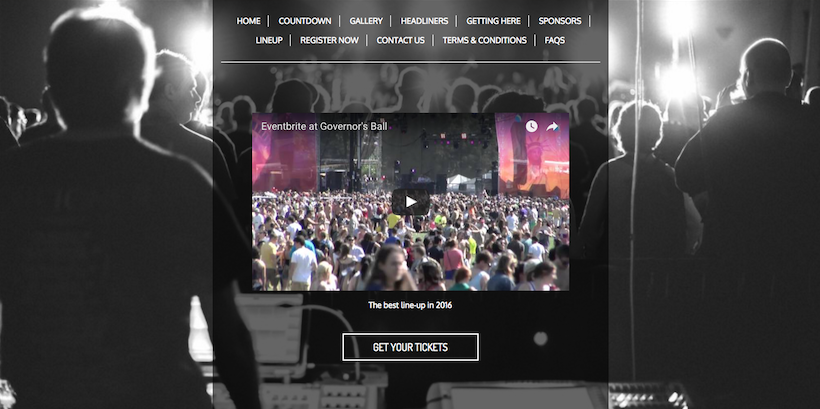The image is a detailed screenshot in black and white, capturing the backs of a crowd of people, illuminated from the front by distant lights. The individuals, dressed in casual attire such as short-sleeved T-shirts, appear to be attendees at a concert or similar event, standing in evenly spaced rows. 

Centrally featured in the image is a text overlay listing menu options: "Home, Countdown, Gallery, Headliners, Getting Here, Sponsors, Line Up, Register Now, Contact Us, Terms and Conditions, and FAQs." Below this, the same backlit crowd appears but in full color, situated in front of what seems to be an outdoor concert stage. 

The vibrant scene depicts an illuminated stage, partially obscured by the silhouetted crowd, who now face the camera. The setting reveals an outdoor venue, enhanced by stage lights and a distant view of the Statue of Liberty to the right, indicating the event's proximity to a prominent landmark. The audience, mostly young adults in their 20s to 30s in casual wear, further solidifies the concert atmosphere.

At the bottom, a highlighted annotation proclaims, "The Best Lineup in 2016," accompanied by a clickable button urging viewers to "Get Your Tickets."